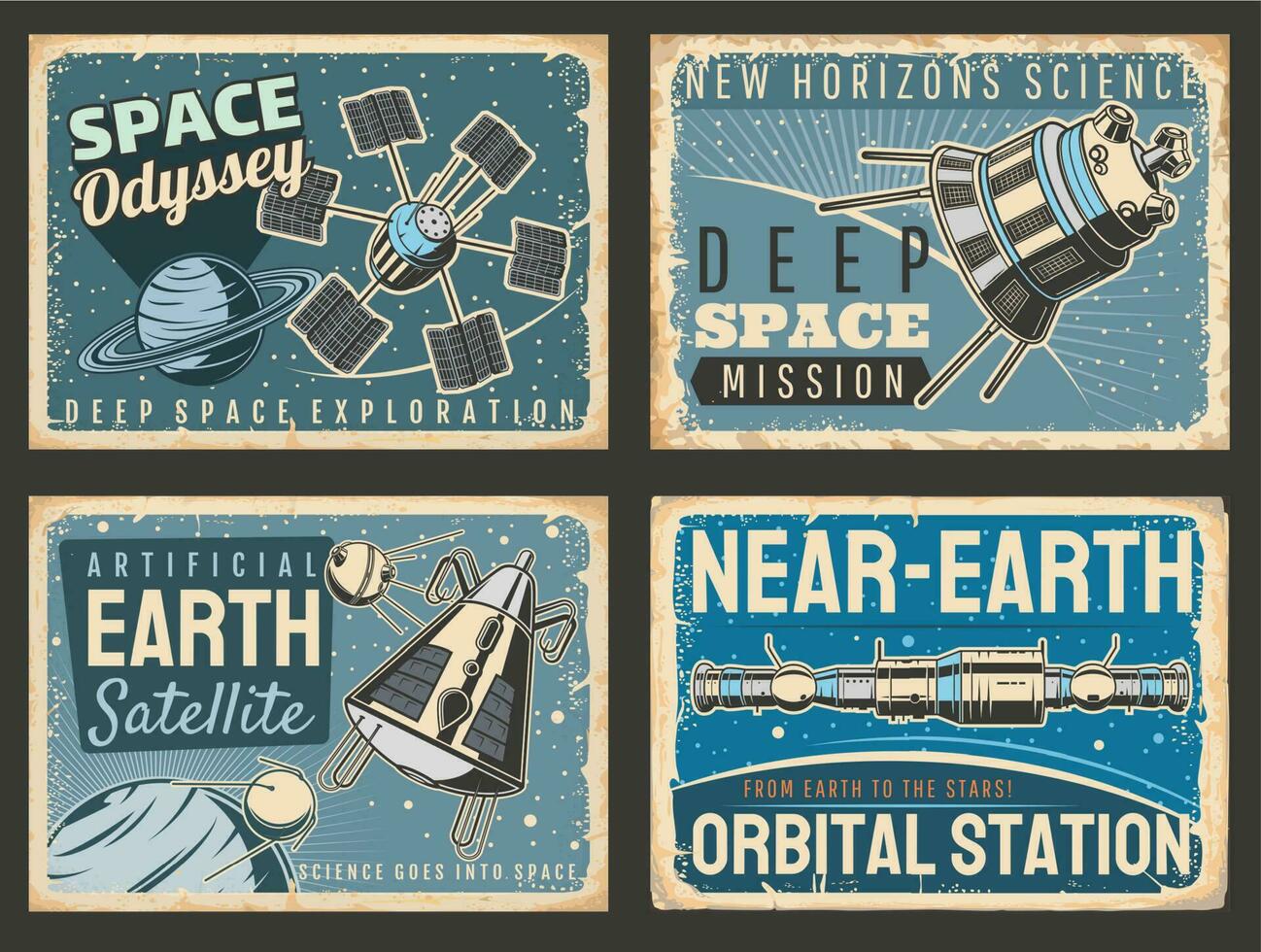The image is a collage of four postcard-sized images, each in a variety of blue, gray, and orange hues, set against a dark gray background with a gray border separating them. Each postcard features a space-related theme. The upper left postcard, predominantly teal blue, showcases a satellite and Saturn, with the titles "Space Odyssey" at the top and "Deep Space Exploration" below. The upper right postcard also in a similar teal blue, features a lunar lander or explorer, labeled "New Horizons Science" and "Deep Space Mission" at the bottom. The bottom left postcard, with another teal blue shade, displays a satellite with the text "Artificial Earth Satellite" at the top and "Science Goes Into Space" beneath it. The bottom right postcard is a brighter blue and highlights a space shuttle or orbital station above a planet, bearing the titles "Near Earth" at the top and "From Earth to the Stars, Orbital Station" at the bottom. Each piece integrates beige text elements, harmonizing the old-fashioned advertisement design with modern space exploration themes.